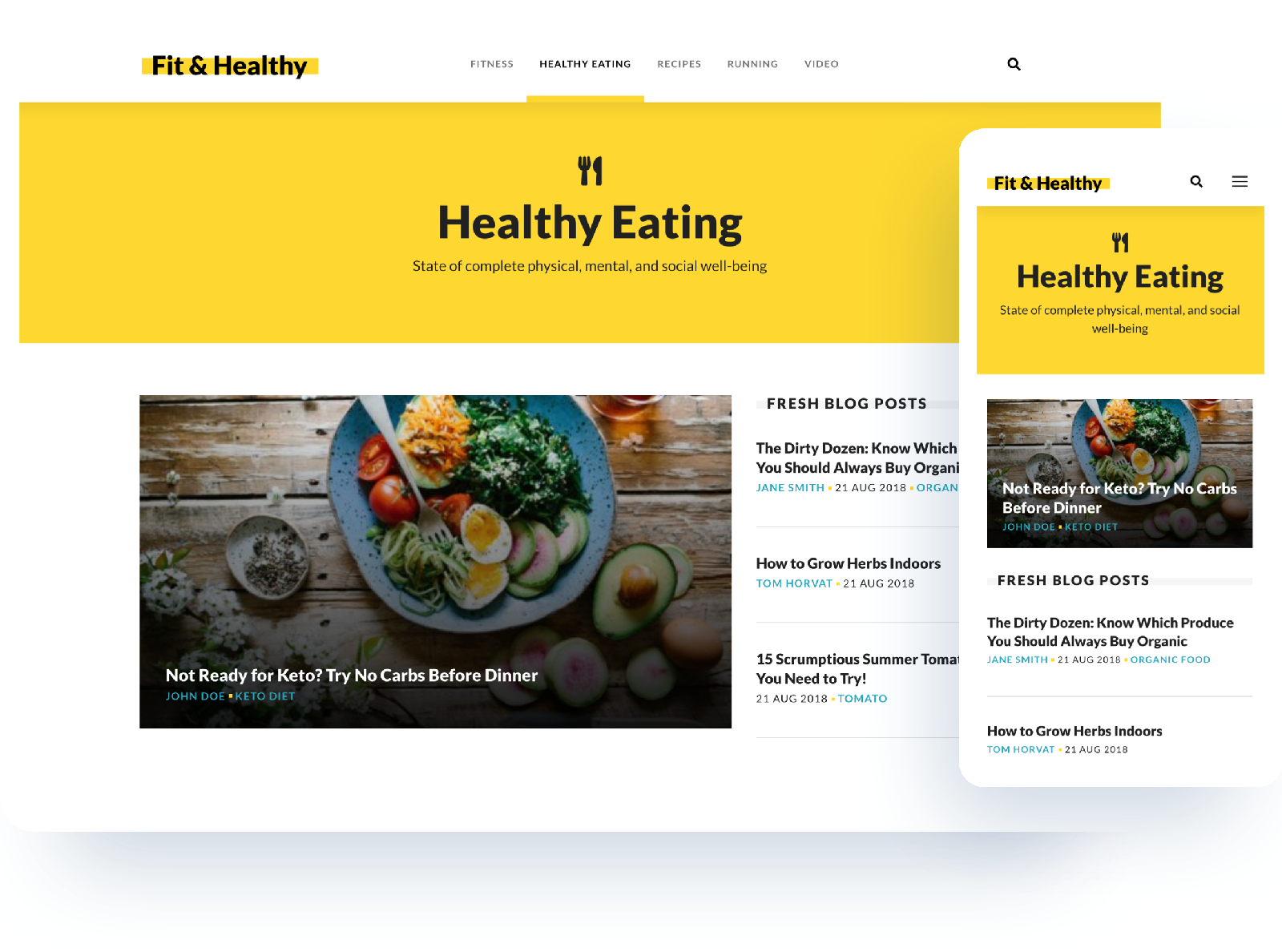The image features a full-size computer screen displaying the website "Fit and Healthy," with a pop-up on the right showcasing how the same webpage appears on a cell phone screen. The pop-up slightly overlaps the computer monitor, emphasizing the responsive design that adapts the content for mobile viewing.

On the larger computer monitor, the background is predominantly white. In the top-left corner, dark bold letters spell "Fit and Healthy," highlighted in yellow. Centralized navigation tabs are labeled with clickable options in gray and black. From left to right, they read: "Fitness" (gray), "Healthy Eating" (black, indicating it is selected), "Recipes" (gray), "Running" (gray), and "Video" (gray), with a black search icon far to the right.

The webpage features a large horizontal bar occupying about a third of the page, with a yellow background and a centered fork and knife icon. Below, in large black letters, it proclaims "Healthy Eating," followed by the tagline "State of Complete Physical, Mental, and Social Well-Being" in smaller black text.

Beneath this section, the screen background transitions to white. The left two-thirds display a photograph of a plate of food on a wooden table. The image features a dish with a fork placed on top, avocados at the bottom right, and another dish to the left. White text across the bottom of the photo reads, "Not Ready for Keto? Try No Carbs Before Dinner," with smaller blue text below identifying the author as "John Doe" followed by a yellow dot and the tags "Keto Diet" in blue.

To the right of the photo, the section is labeled "Fresh Blog Posts" in small dark capital letters. Below, it lists several articles:
1. "The Dirty Dozen – Know Which You Should Always Buy Organic" with author "Jane Smith" in blue, "21 Aug 2018" in gray, and the word "Organ" cut off.
2. "How to Grow Herbs Indoors" by "Tom Horvat" in blue, followed by "21 Aug 2018" in gray.
3. "15 Scrumptious Summer Tomat You Need to Try" with "21 Aug 2018" in smaller letters and "Tomato" in blue; part of the text is cut off by the overlapping cell phone image.

The phone screen replicates elements seen on the computer monitor, including the "Fit and Healthy" header, the "Healthy Eating" pane with its yellow background, and the photograph captioned "Not Ready for Keto? Try No Carbs Before Dinner." It also lists the blog posts "The Dirty Dozen" and "How to Grow Herbs Indoors," but no additional information due to space constraints.